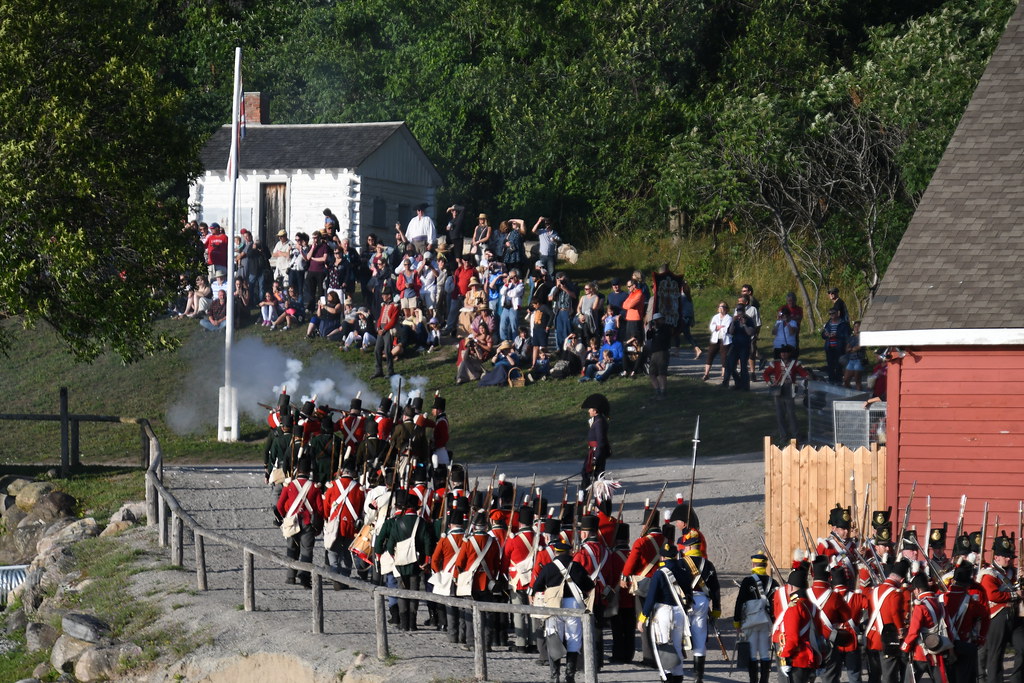The image captures a detailed outdoor scene of a historical war reenactment, likely mimicking a Civil War or colonial battle, featuring a regiment of men dressed as British red coat soldiers. The soldiers are adorned in distinct red uniforms with white cross suspenders, black trousers, and black hats embellished with gold accents, and they are poised carrying muskets with bayonets. The formation is seen marching down a hillside on a gravel path. At the forefront, a smaller group has broken away, actively firing their muskets, creating visible puffs of smoke in the air. Behind them, a crowd of spectators, some taking photos and others shading their eyes from the sun, are gathered on an elevated hillside and along a walkway with railing, observing the event. This crowd is assembled in front of a small white clapboard cottage, which sits against a backdrop of dense forest, suggesting a setting that evokes a historical ambiance, possibly in a historical center or rural town.